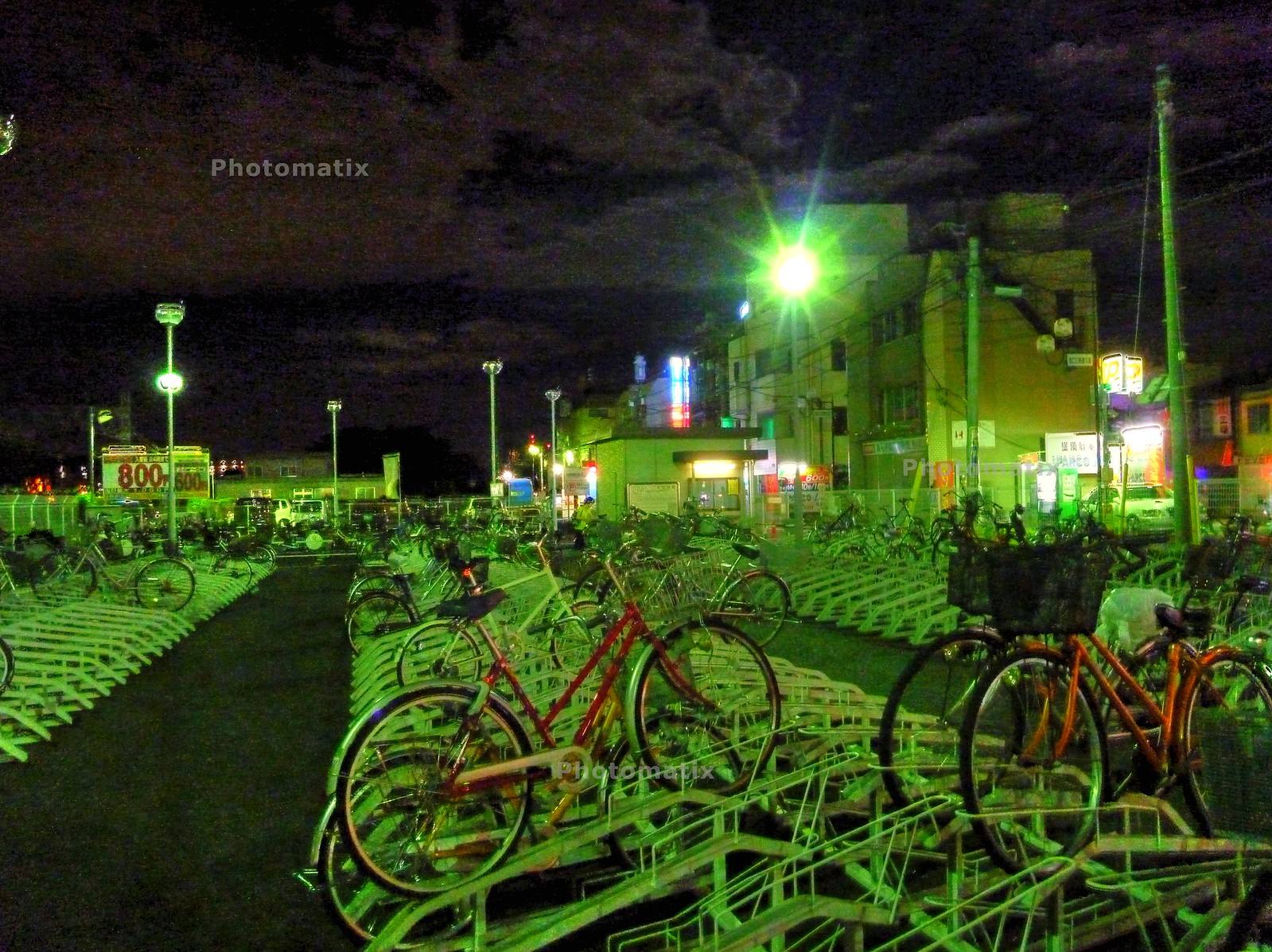The photograph captures a nighttime scene in a bicycle parking lot, dominated by a vivid green glow presumably from a streetlight, which casts a tinted hue over the entire area. The sky above is dark, accentuated by gray clouds, reinforcing the nocturnal setting. The parking lot is filled with ramp-like bike racks, some occupied by bicycles, including those with black baskets on their handlebars, while other racks remain empty. These racks, designed to ease the mounting and dismounting of bikes, start flat, raise slightly, level out, and taper down again. Surrounding the parking area, we can see multiple buildings, some of which bear the numbers "800" and "600," along with power lines and a few streetlights. In the background, cars and trucks are also parked, encased by a chain-link fence that borders the lot. The image distinctly features elements such as the streetlights, power poles, and the false color effect marked by the word "Photomatic" at the top, adding a nostalgic yet surreal tone to the scene.